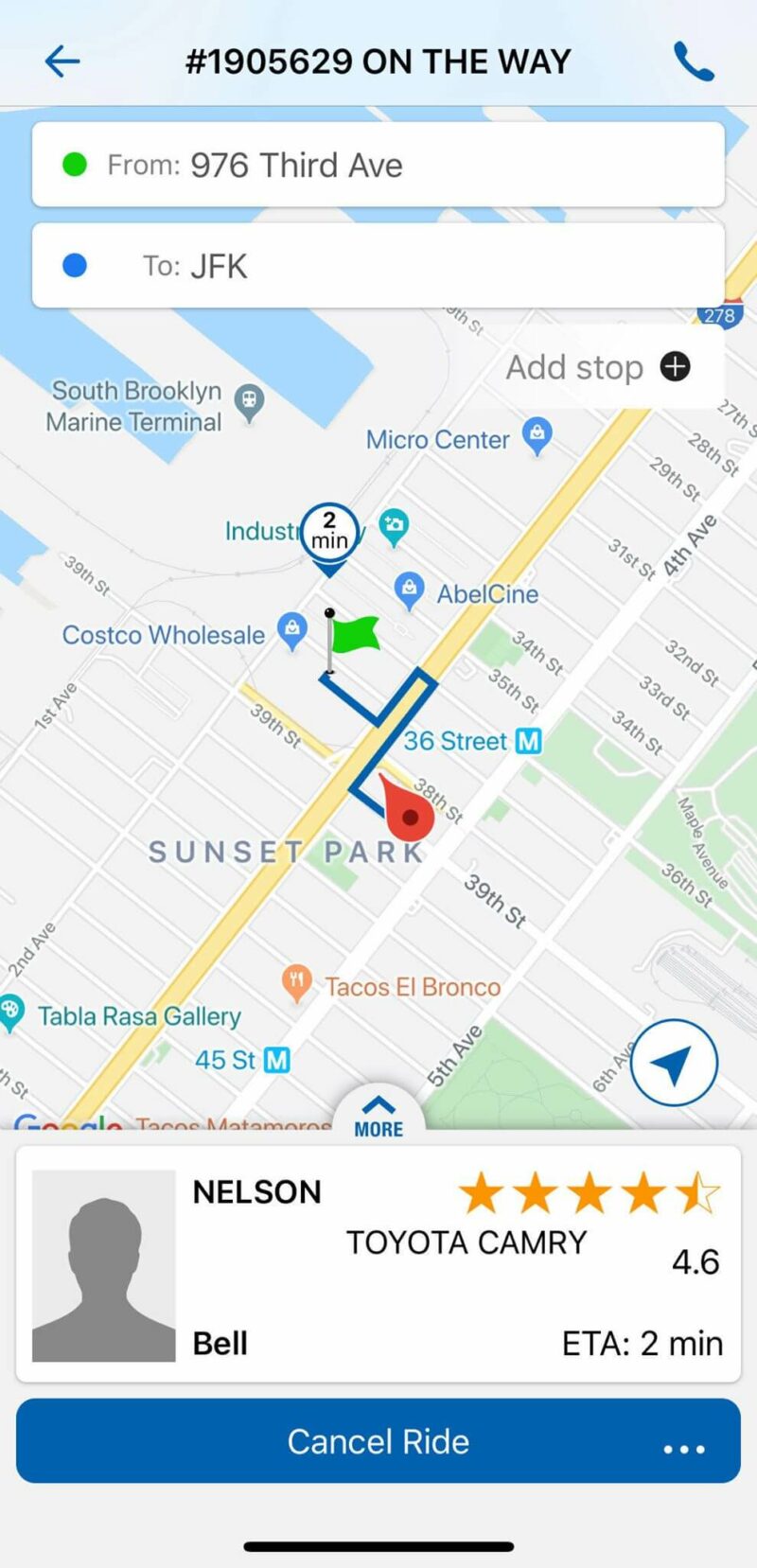The image depicts a screenshot of a ride-hailing app interface against a light blue header at the top. The header displays the text "Pound 1905629 on the way" along with an icon of a blue phone to the right. Below the header, there is a map showing the route and location of the driver. A white information box at the top of the map indicates the pickup location as "From 976 3rd Avenue" and the destination as "To JFK." 

The map itself features a red pin dropped on 36th Street, with notable landmarks such as Sunset Park and a Costco Wholesale visible in the vicinity. 

At the bottom of the map, the driver’s details are presented on a white background: the driver's name is Nelson Bell, and his rating is 4.6 out of 5 stars. The vehicle is identified as a Toyota Camry.